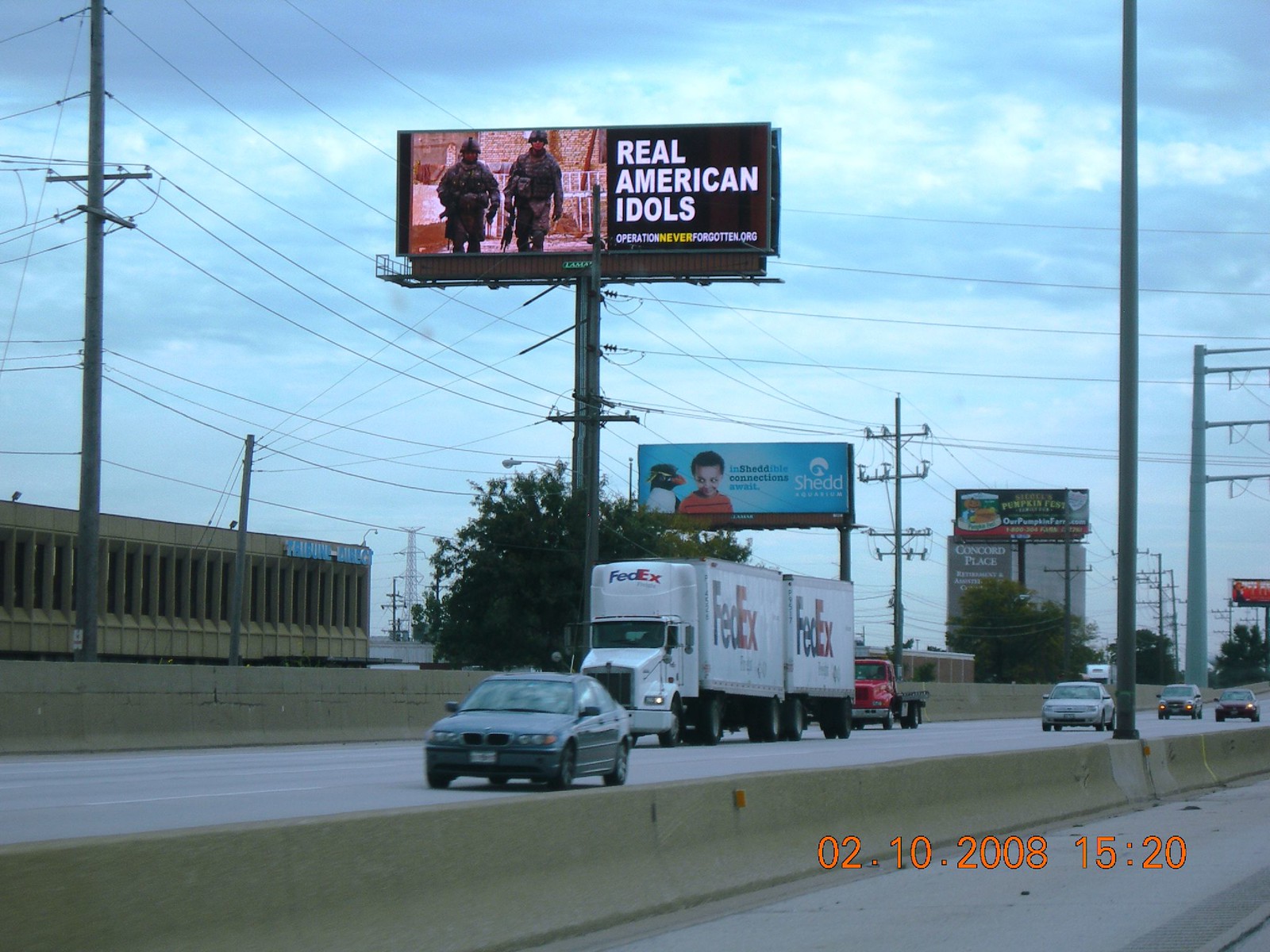A photograph capturing a bustling highway scene on February 10, 2008, at 3:20 PM. The gray-paved highway is divided by an off-white concrete barrier, separating the lanes of traffic. On the highway, a variety of vehicles are visible, including a blue sedan, a couple of white FedEx box trucks, a red truck, and a silver car. The sky above is predominantly blue with scattered clouds. In the background, a prominent black billboard displays the message, "Real American Idols OperationNeverForgotten.org," featuring two individuals in military camouflage fatigues.